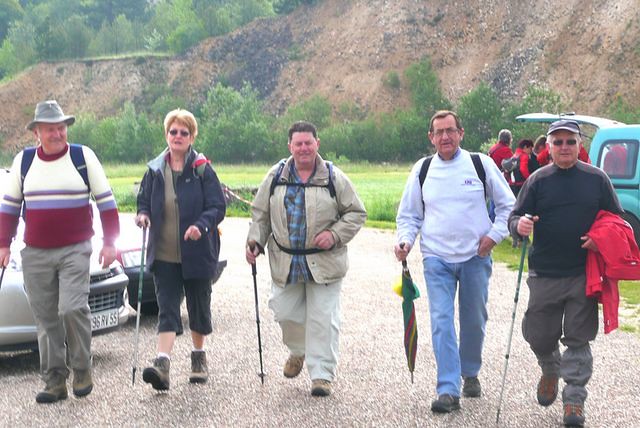The photograph captures five older Caucasian individuals, all wearing hiking attire, walking towards the camera from a parking lot. They are poised for a hike, equipped with hiking poles, apart from one man who is holding an umbrella upside down. On the far left, a man is dressed in a white, red, and periwinkle striped sweater, gray pants, a gray hat, and hiking boots, with a blue-striped book bag on his shoulders. Next to him is a woman in gray boots, white socks, and dark denim shorts; she also is clad in a matching denim jacket. Beside her stands a man in a beige jacket and khaki pants, also prepared for hiking. The fourth person, a man with glasses, is dressed in jeans and a white sweatshirt, carrying a multicolored umbrella. The person on the far right has a long-sleeve black shirt, is holding a red coat, and is equipped with hiking poles. The background reveals a rocky mountainside with green bushes and trees, alongside a parking lot that has several vehicles, including a teal car with its trunk open, where individuals in red attire appear to be preparing for their own hike.